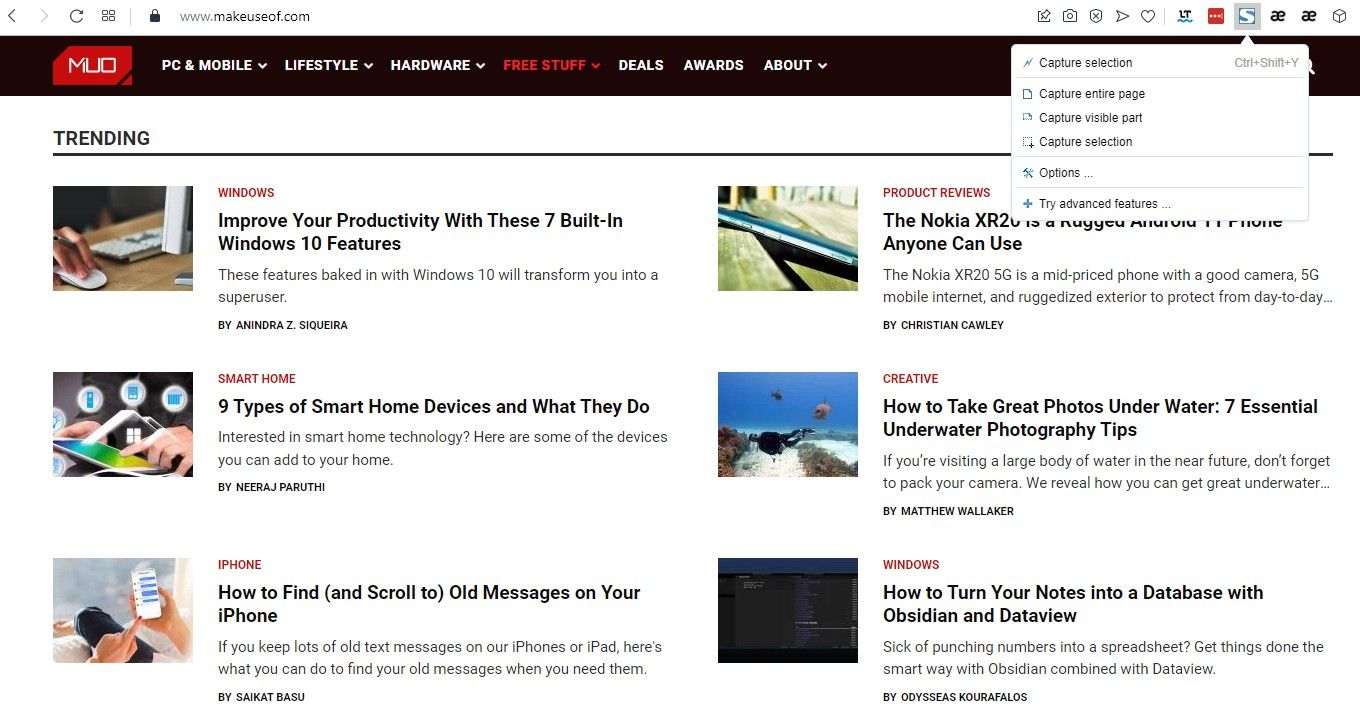This image is a detailed screenshot of a web page from www.makeuseof.com. At the top of the page, the URL is clearly visible. Below it, a dark brown navigation bar spans the width of the page, displaying the site’s logo—a reddish rectangle with the letters "MUD," where the top left and bottom right corners are cut off.

The menu bar beneath the logo contains several categories: PC, Mobile, Lifestyle, Hardware, Free Stuff, Deals, Awards, and About. At the top of the main content area, the word "Trending" is prominently displayed, followed by a horizontal black bar that stretches across the page.

The main section is divided into six articles, organized into two columns with three items each. Each article features a stock image, headline, description, and author’s name. A red tag at the top of each article indicates its category, either "Windows," "Smart Home," or "iPhone."

The first article, categorized under "Windows," is titled "Improve your productivity with these seven built-in Windows 10 features." It details how these features can transform you into a super user, and it is authored by Ninja Zekera.

The second article falls under "Smart Home" and is titled "Nine types of smart home devices and what they do." It offers insights into various smart home technologies and how to integrate them into your home, written by Neeraj Paruthi.

The third article is in the "iPhone" category and is titled "How to find and scroll to old messages on your iPhone." It guides users on finding old messages on their iPhone or iPad, authored by Sycat Basu.

The description for the fourth article, under "Product Reviews" and related to the Nokia phone, is cut off in the provided text. Each article is clearly structured to provide users with informative content relevant to their interests and needs.